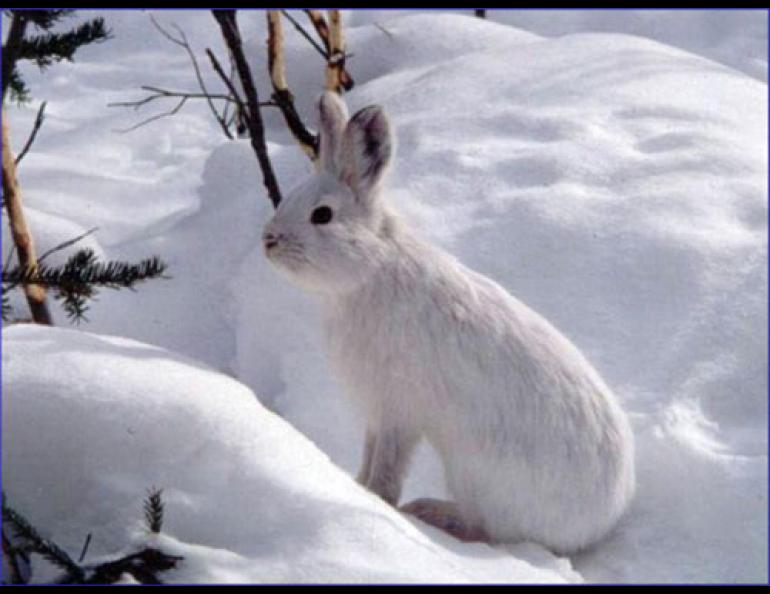The image captures an outdoor winter scene, possibly a screen capture from a video, as indicated by the blue border encircling it with a thicker black border along the top and bottom. Set against a backdrop of untouched, pristine snow, the focal point is a white snowshoe rabbit sitting in the center, surrounded by snowdrifts. The rabbit, with distinctive black-tipped ears and black eyes, is poised on its hind legs, gazing to the left as if sensing something. Behind it, tree branches and barren limbs from a small bush emerge from the snowdrift. To the right, evergreen branches with snow-covered bristles stick out, suggesting part of the tree is embedded in the snowdrift. The scene is illuminated by sunlight from above, casting a serene and tranquil ambiance over the winter landscape.